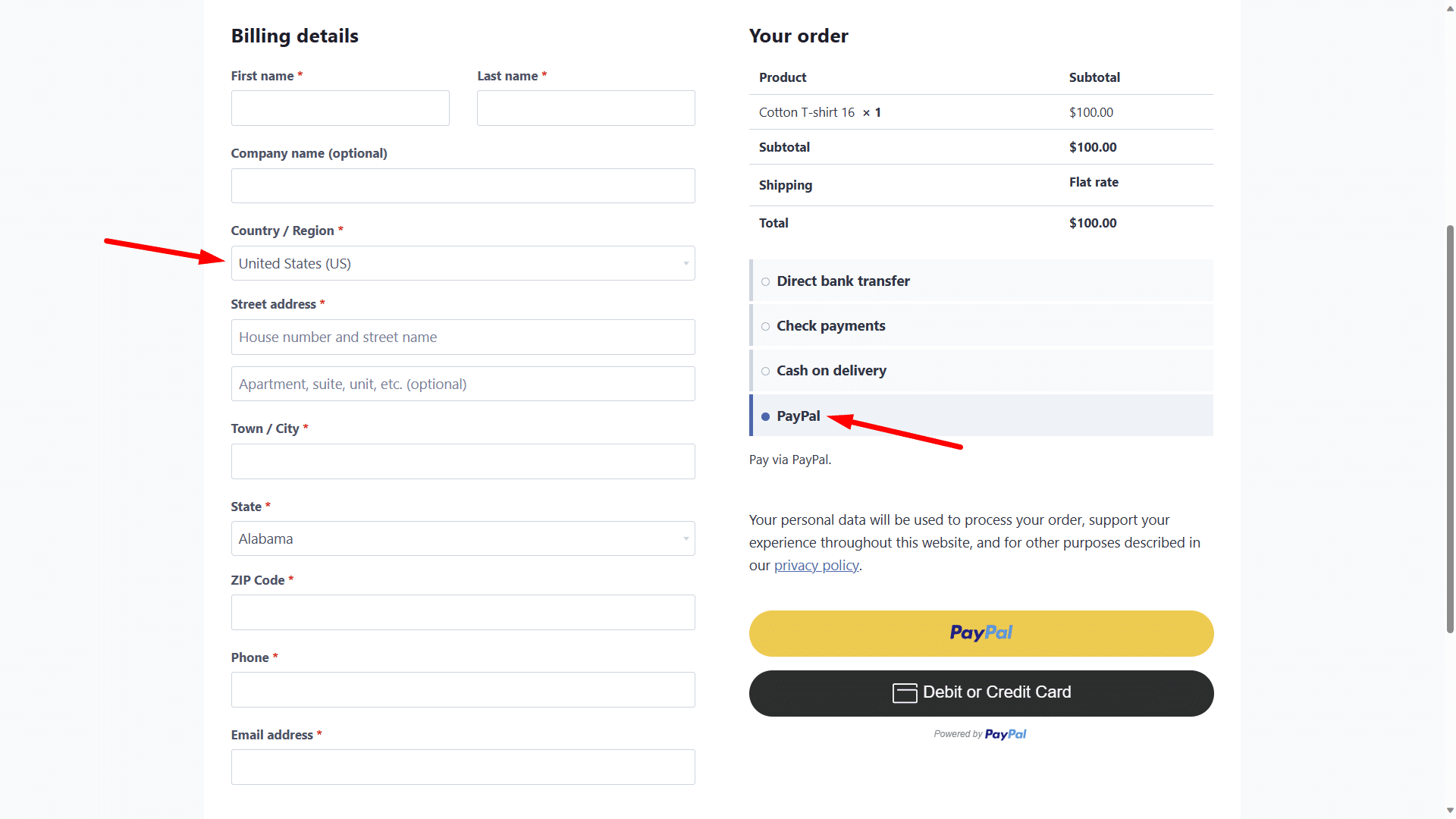The image appears to be a screenshot from a mobile website displaying the billing details section of an online purchase form. The layout shows two distinct sections: one for inputting personal details and another summarizing the order.

At the top of the image, the text "Billing Details" is prominently displayed. Below this header, fields for inputting information such as "First Name," "Last Name," and "Company Name (optional)" are clearly visible. A dropdown menu labeled "Country/Region" shows "United States (US)" as the selected country. A red arrow points from left to right, emphasizing the "United States."

The lower section of the image, which details the order summary, shows a PayPal payment button highlighted by another red arrow pointing to it from the right. The order summary outlines a purchase of a "Cotton T-Shirt," with a quantity of 1, priced at $100. The total amount listed for the order is $100, with flat-rate shipping fees mentioned but not specified. The total bill reads "$100."

Payment options listed include "Direct Bank Transfer," "Check Payments," and "Cash on Delivery," with "PayPal" selected.